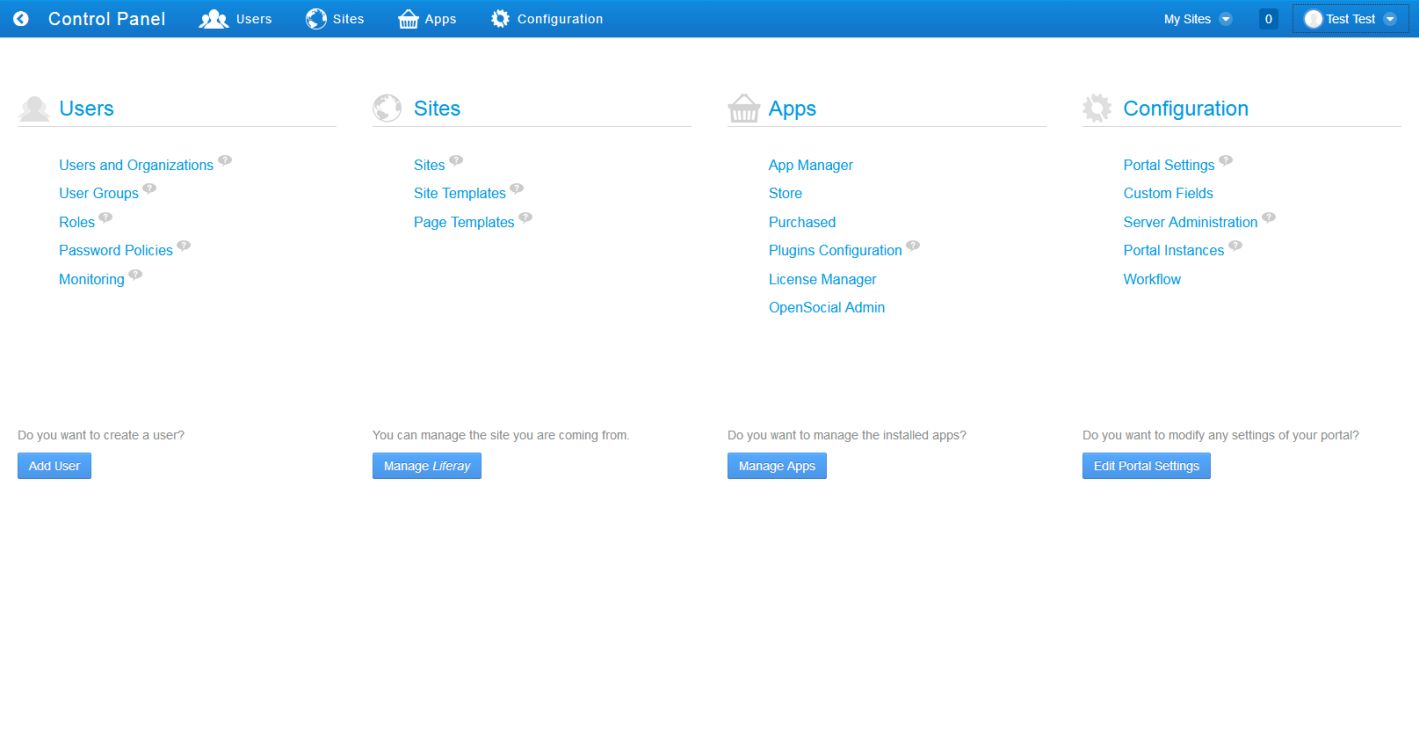The image features a control panel interface that is approximately two to three times wider than it is tall. The upper section of the image, occupying around 10-15% of its height, is a blue bar extending from left to right. This bar includes several white icons and text: a left arrow, the words "Control Panel," an icon of three silhouettes labeled "Users," a globe labeled "Sites," a shopping basket labeled "Apps," and a gear labeled "Configuration." On the far right side of the bar, it reads "My Sites" with a down arrow beside it, followed by a "0," and a dropdown box containing the text "test."

The lower, main section of the interface has a white background and displays four main categories horizontally listed with their corresponding icons: "Users," "Sites," "Apps," and "Configuration," mirroring the items found in the blue bar above. 

Beneath these headers, each category contains specific links:
- Users: Five different links with the text "Do you want to create a user?" at the very bottom, accompanied by a blue button saying "Add User."
- Sites: Three links followed by a button with a contextually appropriate action.
- Apps: Six links, also ending with a category-specific button.
- Configuration: Five links, culminating in another unique button related to its category.

Each button at the bottom of these sections has white text that indicates its action, matching the interface's clean and organized design.